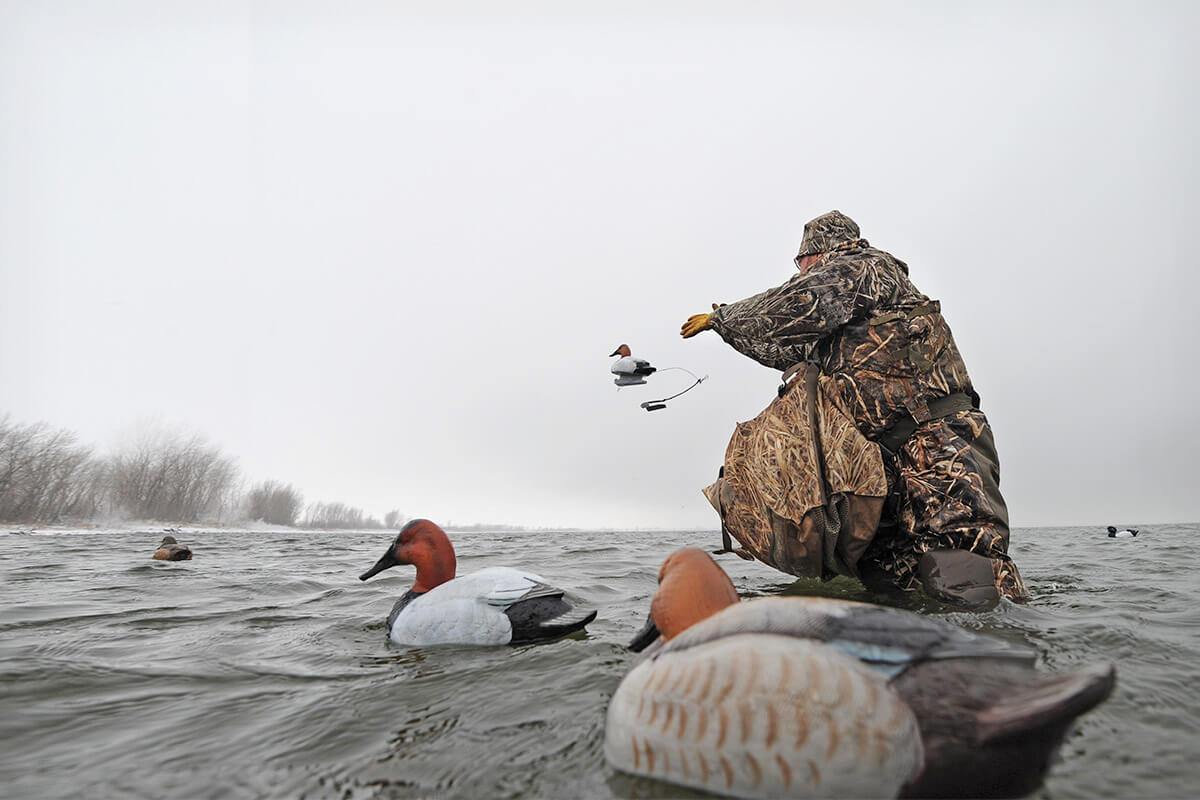The photograph showcases a winter scene with a hunter in full camouflage gear wading in the gray, choppy waters of a lake. Framed in a low-angle shot, the viewer's eye is drawn to the hunter, who is clad in camouflage patterns that blend seamlessly into the surrounding environment. The hunter, wearing beige and dark green camouflage, including a hat and wading pants, is positioned on the right side of the image, facing left. He is throwing duck decoys into the lake, reaching into a large camouflage bag slung over his shoulder. The decoys, scattered around him in the water, have distinct red heads, white wings, and black bodies, with some variations having orange heads and black feathers. The water stretches to the horizon, under a grayish-blue, cloudy winter sky. The distant shoreline on the left bears the stark, leafless silhouettes of trees against a backdrop dusted with snow. The scene is serene and meticulously detailed, capturing the essence of a winter hunting expedition.